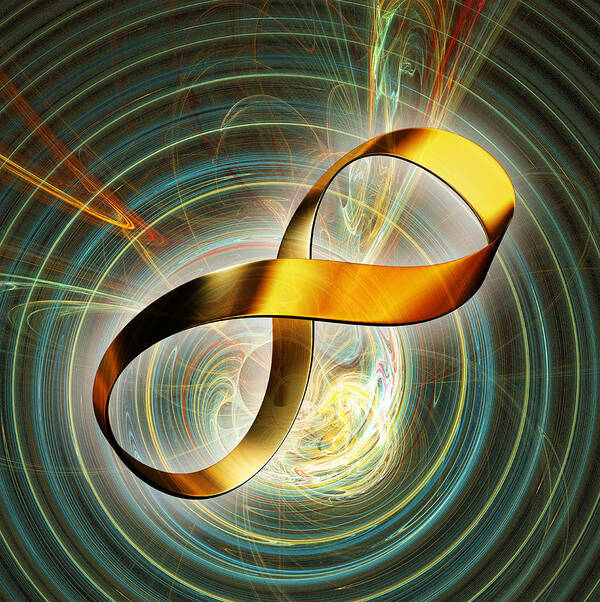This digital image, likely created using a computer program, depicts a striking and intricate scene of light and shapes. At the center of the composition, there is a large, metallic gold infinity symbol or Möbius strip, which shines with well-defined highlights and contrasts, giving it a reflective and glossy appearance. The symbol is positioned diagonally, evoking both the infinity symbol and a figure-eight pattern.

Surrounding the golden figure are concentric circles of thin bands of light, reminiscent of illuminated objects spun on a turntable. These bands alternate between blue and a green-yellow hue, creating a striped effect. 

Adding to the complexity, there is a dynamic and organic swirl of colors—orange, red, green, and yellow—that emanates outwards from the center. This fluid light, appearing almost as if it is moving in slow motion, forms occasionally tangled and messy sections. These colorful swirls contribute to the image's overall sense of energy and movement.

The background is a rich tapestry of digital effects, including laser-like beams and long exposure light trails. These lights predominantly feature green and blue tones, with occasional bursts of orange. The entire scene has an early internet graphic aesthetic, marked by a sense of vibrant, swirling energy and glowy bits of light scattered throughout.